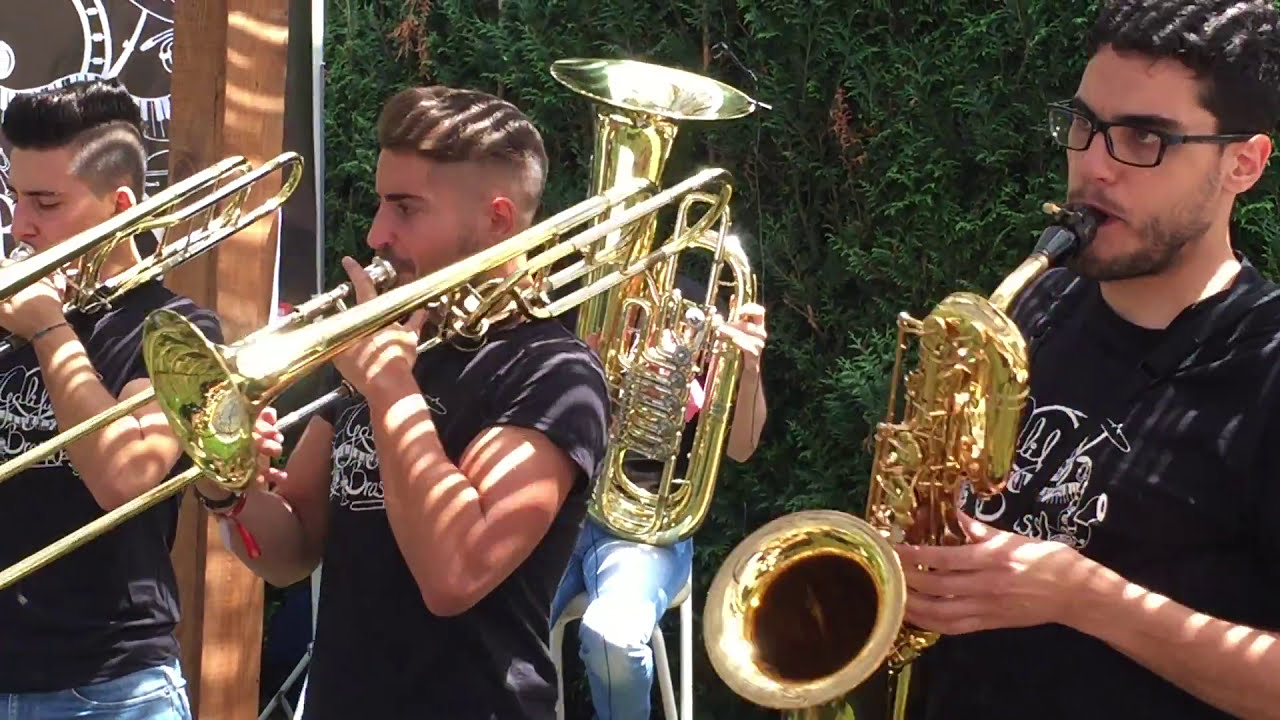The image captures an outdoor ensemble of four musicians with intricate details. On the far left, partially cut off, is a man with short black spiky hair, wearing a black t-shirt and blue jeans, playing a trombone. To his right stands another trombone player, distinguishable by his short brown hair and black t-shirt with white illustrations. Both trombones glisten with reflections from their brass surfaces. In the background, partially obscured, is a seated individual holding a tuba, with only their blue-jeaned legs and left arm visible around the instrument. On the far right stands a man with black hair, black glasses, a bit of a beard, and a matching black and white t-shirt, playing a baritone saxophone, his left hand positioned on the keys. The scene's backdrop is filled with dense greenery, including trees, bushes, and a wooden column, highlighted by the natural sunlight casting shadows and glares. The musicians are angled slightly to the left, creating a dynamic and engaging composition.